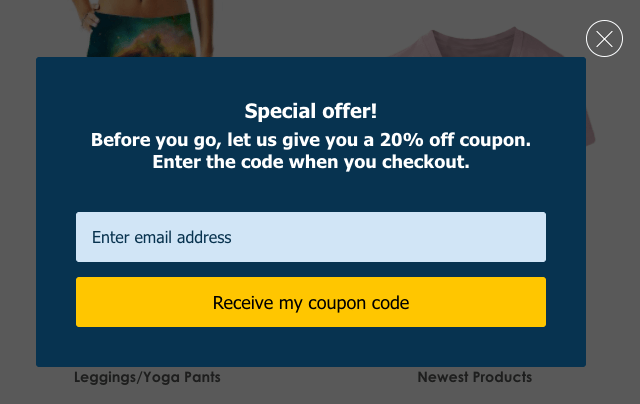The image showcases a promotional overlay on a grayish background. Dominating the center is a blue rectangular box bearing the phrase "Special Offer!" at the top, accompanied by a circle with an 'X' in it, possibly indicating a close button. Below "Special Offer," the text "Before you go, let us give you a 20% off coupon." is centrally aligned. The call to action beneath instructs users to enter a code during checkout for the discount.

Beneath this, two input fields with rounded edges and uniform length are present. The upper input field is a light gray color, prompting users to "Enter email address." The lower input field is strikingly yellow and read "Receive my coupon code" in its center.

On the left side of the image, there is a smaller box featuring a child with hands on hips, dressed in rainbow-patterned shorts. Below this box, the text "Leggings/Yoga Pants" is visible. At the bottom, a banner with the title "Newest Products" appears alongside a partially visible image of a pink V-neck shirt, cut off just above the shoulders.